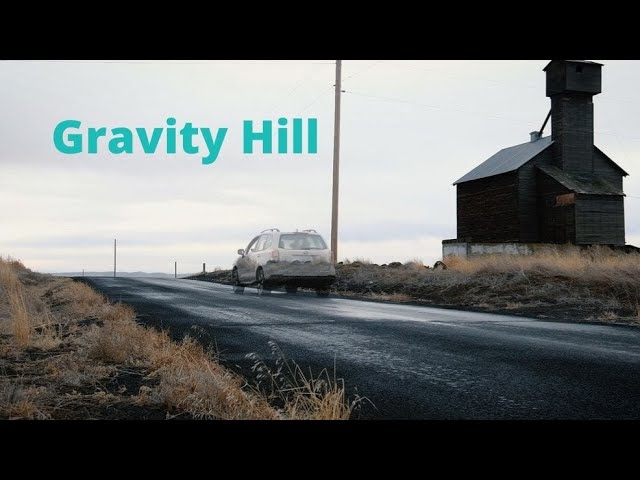The image captures a countryside scene featuring a narrow, dark asphalt road that stretches through the center. Prominently placed in the center of the image is a small, tannish SUV, with a peculiar semi-transparent quality that makes its tires nearly see-through. The road appears recently wet, adding a dark sheen to its surface. On the top left of the photo, the phrase "Gravity Hill" is clearly visible in green lettering against a gray, cloud-streaked sky. Flanking the road on both sides, the landscape is composed of yellowish, dry grass interspersed with greenish-yellow weeds. To the right of the car stands an old, black barn, with an appearance suggesting it was once used for storing grain or seeds. The entire photograph is letterboxed with black bands at the top and bottom, framing the rustic, slightly eerie countryside setting.